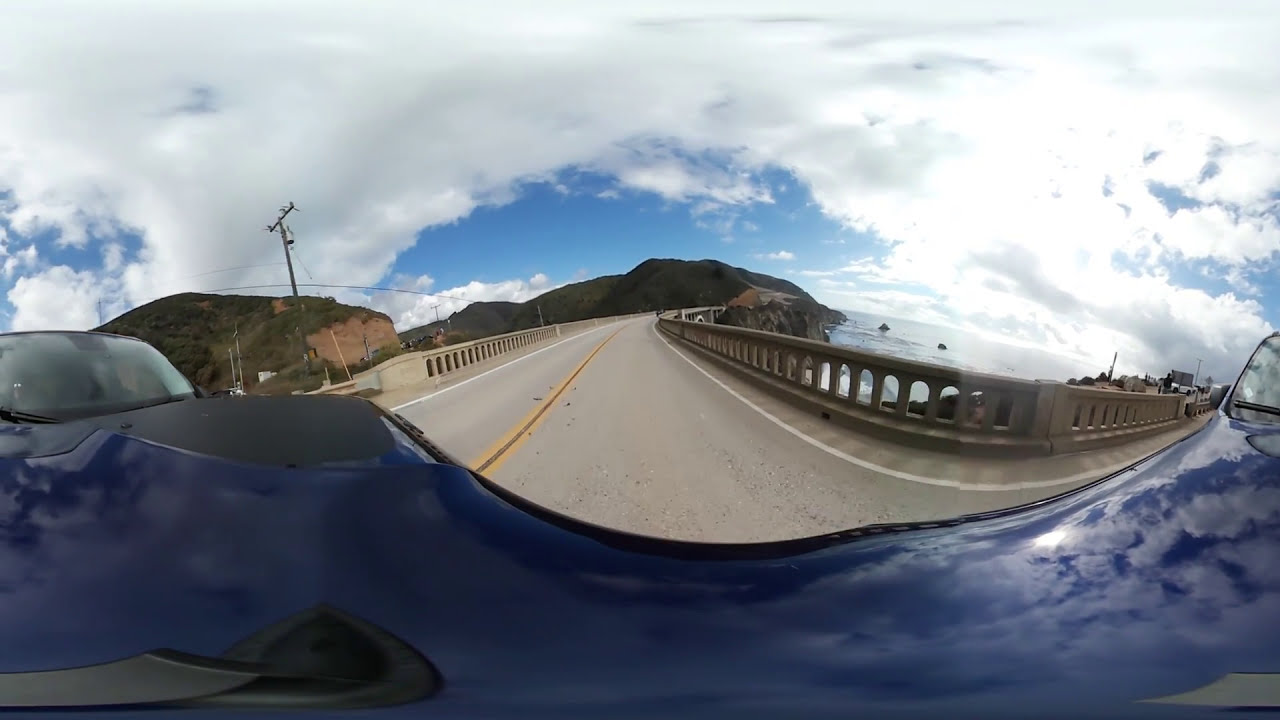The image captures a stunning fisheye lens perspective, likely from a dash cam, looking down a roadway traversing a bridge, with significant distortion. At the bottom of the frame, the blue hood of a car is visible, reflecting the clouds and sunlight on the right side, while exhibiting a foggy glass bulge on the left. The asphalt road ahead is a light gray, marked with double yellow lines in the center and white lines on the sides. The bridge features flat-topped concrete barriers with visible arches beneath them. Midway down the bridge, people can be seen standing on the wrong side of the barrier. To the right, light reflects off a distant body of water, possibly the ocean. On the left, there is a light orange cliff with green vegetation atop the mountains and a power line tilted towards the left. The sky is predominantly cloudy with dark gray clouds on the left and brighter, sunlit clouds on the right, framing a patch of blue sky in the center. The overall scene suggests a picturesque, possibly Hawaiian, landscape on a bright summer day, highlighting both natural beauty and man-made structures.